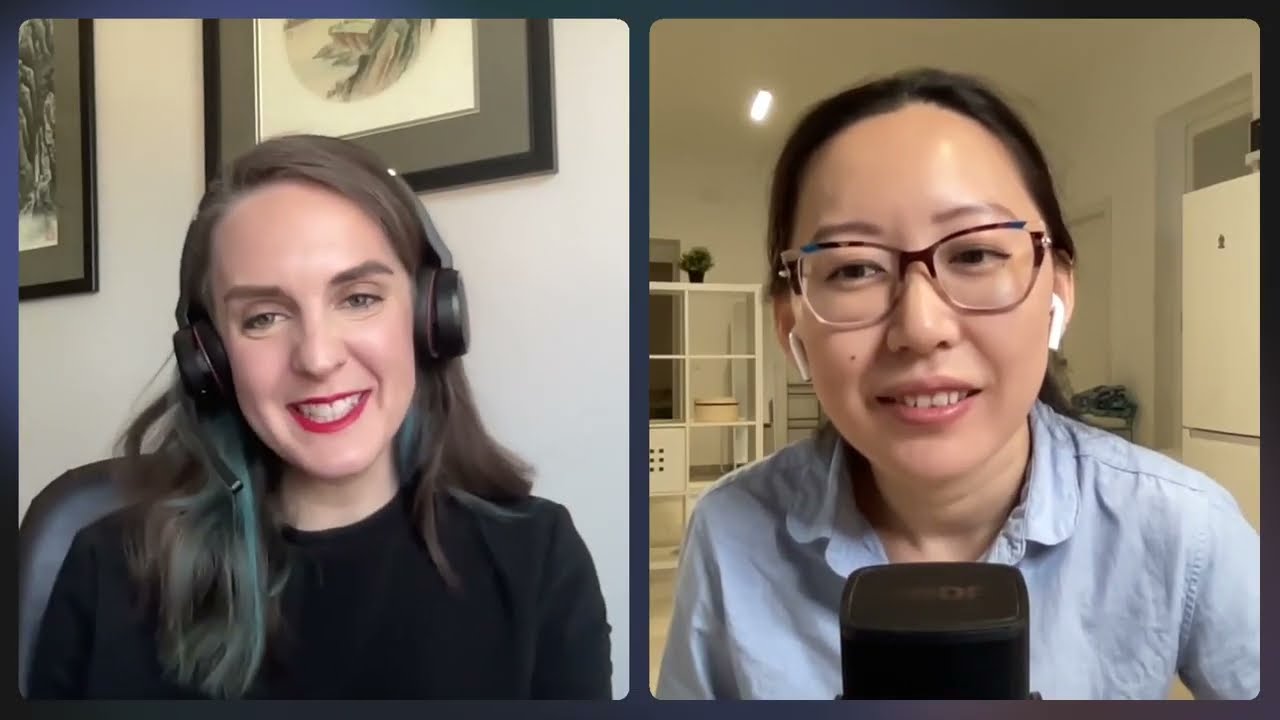This image depicts a video call between two women, with the screen split in half to show each participant. On the left is a Caucasian woman with long, brownish hair, wearing over-the-ear headphones and a black, round-necked blouse. She is smiling broadly, highlighting her red lipstick, while seated on a dark or leather chair. Behind her is a white wall adorned with two framed pictures.

To the right is an Asian woman with glasses and brown hair combed back, wearing iPod earbuds and a blue, open-collared shirt. She has a slight smile and appears to be conversing into a microphone. Her background reveals an apartment setting, featuring a refrigerator, shelves with some pottery, cabinets, and a plant above her left shoulder. Both women are looking directly at the screen, indicating they are engaged in a conversation, likely on a Zoom call.